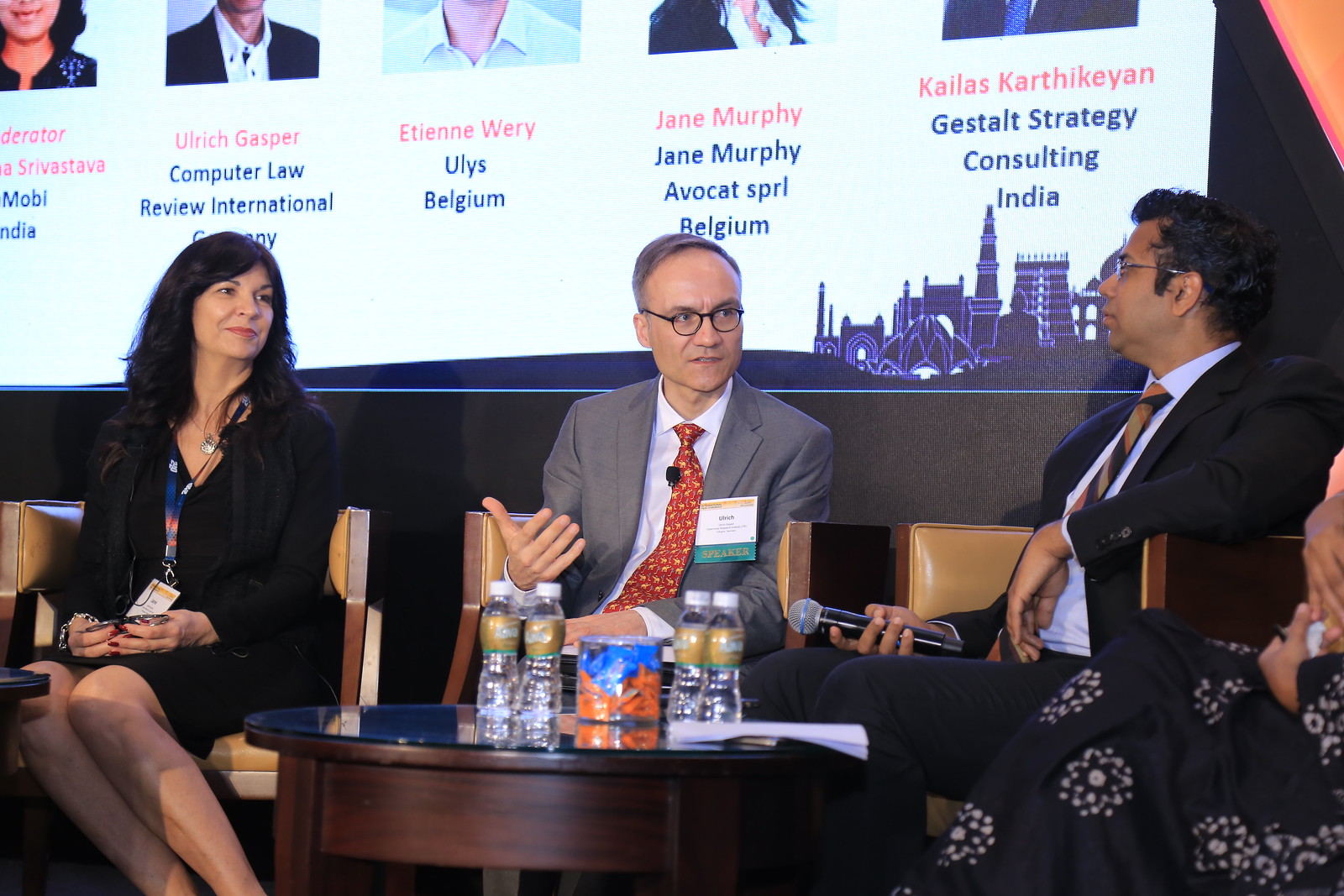The image captures a panel discussion at a conference or television recording, featuring four participants dressed in professional attire. To the left, a woman in a black suit, adorned with a lanyard and pass, directs her focus to the two men seated beside her. Central to the scene is a gray-haired man in a gray suit, white shirt, and red tie, who actively gestures with his right hand while speaking, thanks to a microphone clipped to his tie. Beside him, another man, outfitted in a dark suit, glasses, and a striped tie, holds a microphone in his lap. On the far right, only the lower half of another woman is visible, distinguished by a dark skirt with a white pattern. 

In front of the panelists is an oval coffee table bearing four water bottles, a jar of snacks, and some papers. A screen behind them displays partial images and names of individuals involved in the event, including Ulrich Gaspar from the Computer Law Review International, Germany; Etienne Berry from Ulysse, Belgium; Jane Murphy from SPRL, Belgium; and Kailash Karthikeyan from Gestalt Strategy Consulting, India. Additionally, a "City Line" logo appears on the lower right corner of the screen.